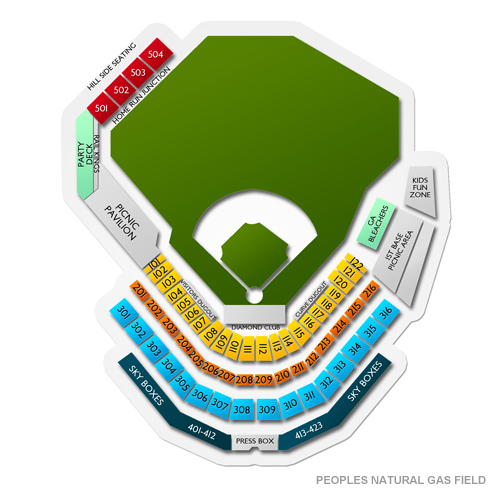The image depicts an overhead view of an outdoor amphitheater, complete with detailed seating arrangements and various amenities. The amphitheater features multiple sections, each with distinct color-coded seating. The front-facing section has a row of seats numbered 101 to 122 in yellow, the next row up is numbered 201 to 216 in orange, followed by a row numbered 301 to 316 in blue. Beyond these rows are the skyboxes, covering seats 401 to 423.

Surrounding the seating areas, you will find several picnic pavilions, party decks, and additional picnic areas, as well as a kids' fun zone. These amenities are spread out around the edges of the amphitheater. The main central area is a large green space, with a particularly expansive back portion. There is a noticeable white gap within this green area, followed by another central green section.

In the top left corner of the image, hillside seating is provided for seat numbers 501 to 504, which are colored red. The entire layout is meticulously organized to cater to various needs, offering a comprehensive view of the seating and surrounding facilities.